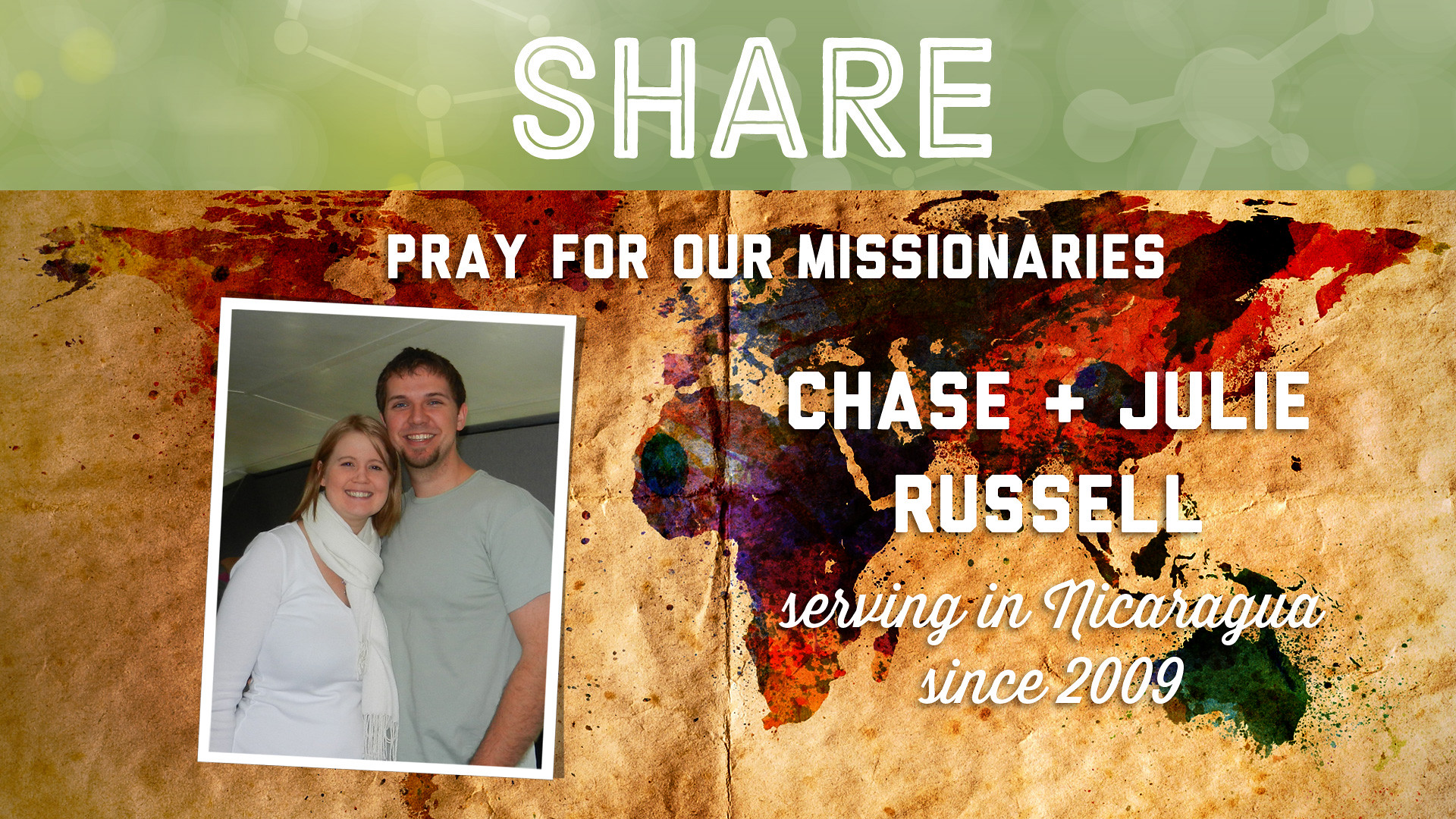The image features a top section with a greenish-gray stripe that displays the word "SHARE" in bold, white letters. Below this, the background transitions to a brown area with an aged, paper-like texture featuring a colorful map where the countries are depicted with paint splatters in dark hues like purple, green, and red. A noticeable crease runs down the middle of this section, suggesting it might have been folded. Centered in large, white, capital letters, it reads "PRAY FOR OUR MISSIONARIES." To the right, the text continues with "CHASE + JULIE RUSSELL" and in a script font beneath, "SERVING IN NICARAGUA SINCE 2009." On the left side, there is a photograph of a smiling couple: the woman with light-colored hair, wearing a white long-sleeved top and a white scarf; and the man, with short brown hair and a beard, dressed in a light green shirt.